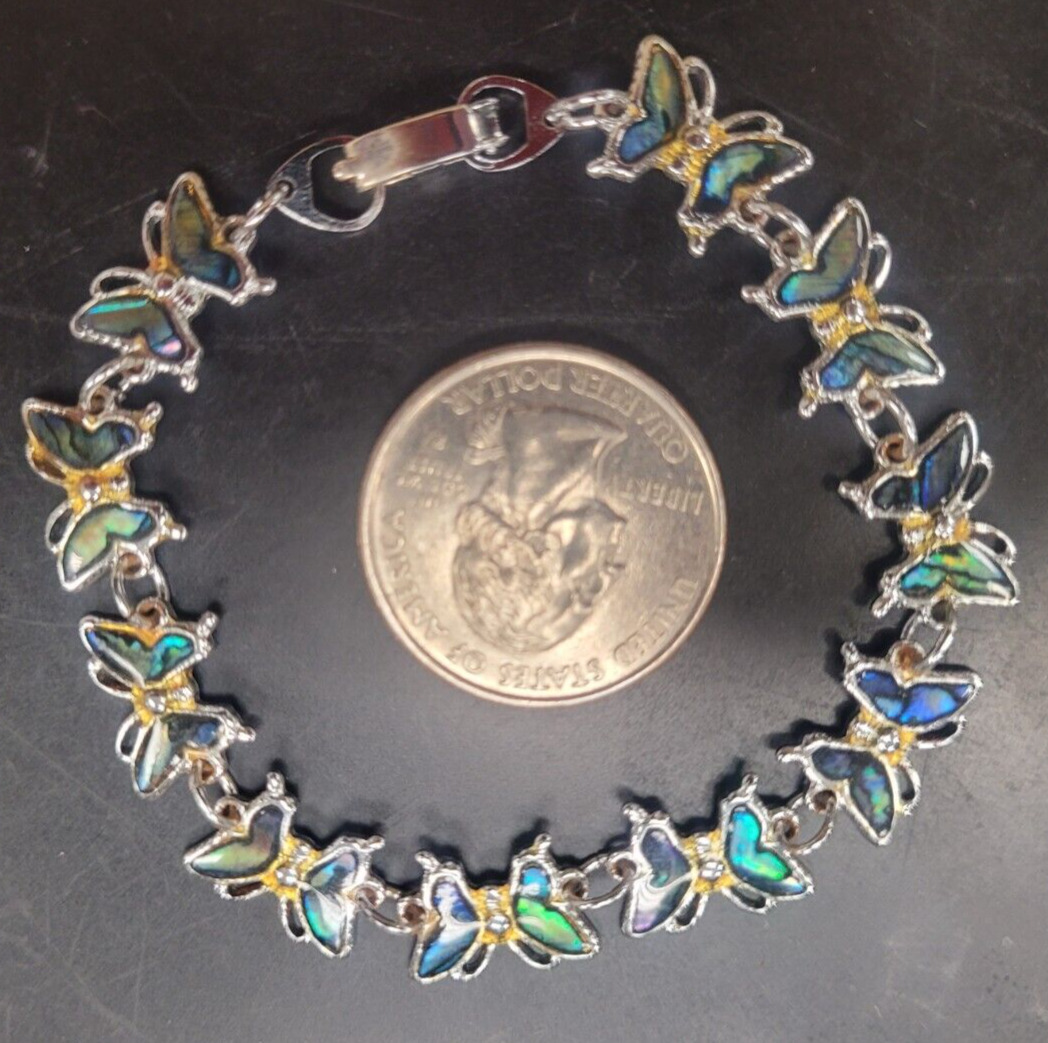This detailed photographic image, captured from an overhead perspective indoors, showcases an intricate golden bracelet, composed of approximately 15 butterfly charms, encircling an upside-down Washington quarter. The butterflies feature vibrant wings in hues of greenish-blue, green-grey, blue, and predominantly green and blue combinations, adding a landscape of color to the otherwise grey and slightly marked surface on which they rest. The quarter, centrally placed and shining due to the camera flash reflection, bears the inscriptions "United States of America," "Liberty," and "In God We Trust," typical of a US quarter dollar. The size reference provided by the quarter underscores the bracelet's delicate and possibly child-sized dimensions, with minimal space—about half an inch—surrounding the quarter within the circular arrangement of the butterflies.